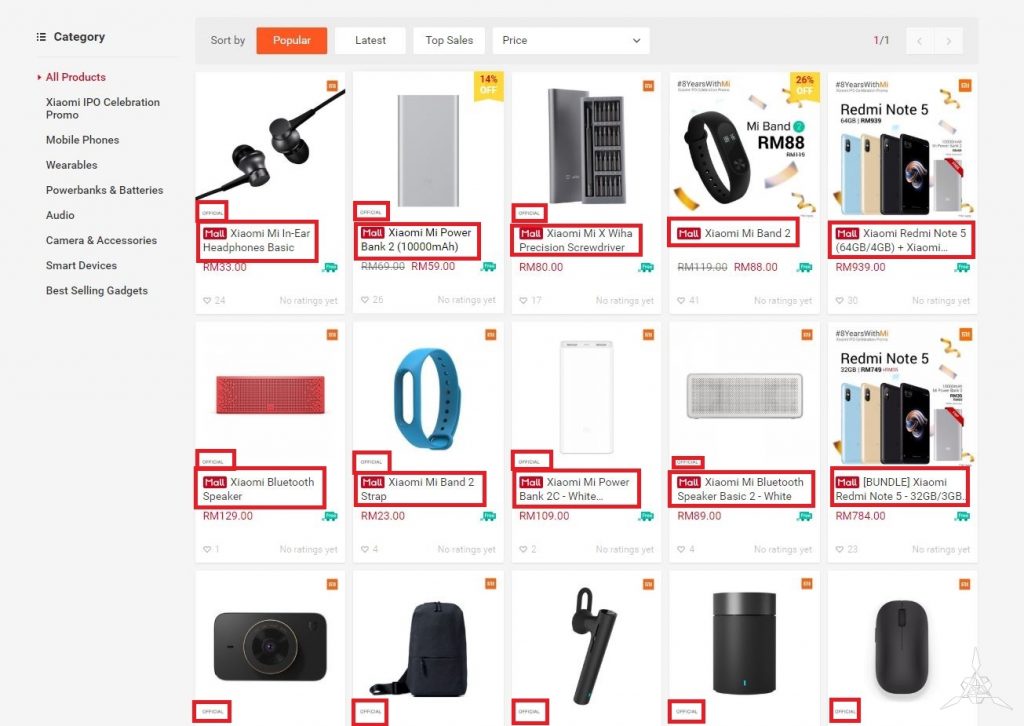The image depicts a shopping website interface. On the left side of the screen, there is a category menu. At the top left, in black text, there is the heading "Categories". Below this, in red text, it says "All Products". Following this, in black text, is an extensive list of product categories such as "XIAOMIIPO Celebration Promo", "Mobile Phones", "Wearables", "Power Banks and Batteries", "Audio", "Camera and Accessories", "Smart Devices", and "Best-selling Gadgets".

On the right side of the screen, the main page displays various products available for sale. At the top of this section, there are sorting options: "Popular", "Latest", "Top Sales", and "Price". The sorting option "Popular" is currently selected, indicated by an orange highlight, whereas the other options remain with white backgrounds.

Underneath the sorting options, there is a grid of product listings. These include items such as headphones, watches, cell phones, Bluetooth speakers, and wristbands. Each product image is accompanied by a product title outlined with a red rectangle. The prices of the products are also displayed prominently, with prices marked in Malaysian Ringgit (RM), such as RM 784 or RM 89.